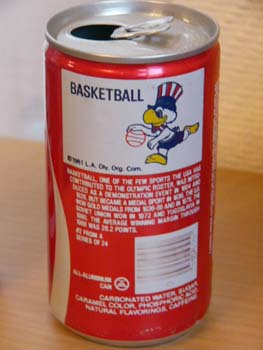The image is a close-up color photograph in portrait orientation featuring an opened soda can, resembling a Coca-Cola can. The silver top of the can, complete with the familiar pull-tab that has been pressed down to reveal the black circle of the can's opening, dominates the image. The can's body is predominantly red with a distinctive white stripe running down the left-hand side, tapering at the top, curving slightly to the right before extending straight downwards—indicative of Coca-Cola's stylized branding. 

On the upper portion of the can's back, a white rectangle with the word "BASKETBALL" inscribed in bold, black capital letters on the left is prominently displayed. Next to this text, an anthropomorphized duck with a yellow beak—possibly a reference to a special or limited edition promotion—illustrates the theme. This duck, engaged in playing basketball, wears an American-style hat featuring a navy band with red and white vertical stripes, suggesting a connection to an American basketball event or team. The basketball is depicted in a red outline. 

Additional details include a list of ingredients and a barcode located at the bottom right corner of the can, set against the red background with white text. This intricate design implies the can was released as part of a special campaign celebrating basketball.